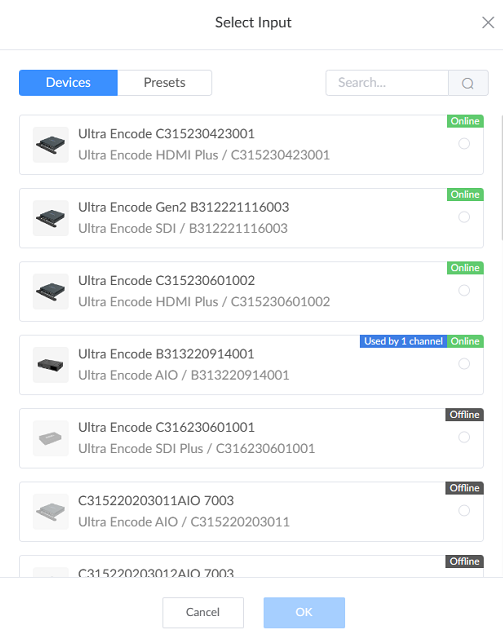This is a detailed screenshot of a user interface, likely from a software application. At the top center of the screenshot, there is a header labeled "Select Input." On the upper right corner, there is an "X" icon, presumably for closing the window. Below this header, a horizontal gray line separates it from the main interface.

The main section is divided into two tabs: on the left half, there is a blue-filled box labeled "Devices" in white text, and on the right half, a white box labeled "Presets" in black text. To the right of these tabs is a small gray search box featuring a gray magnifying glass icon inside.

Underneath this main section, there is a list of devices, each contained within a gray box. The first device in the list has an image that appears to be a hard drive. It is labeled "Ultra Encode C315230423001" in black text, with a smaller gray text below that reads "Ultra Encode HDMI Plus / C315230423001." In the upper right corner of this gray box, a green box with the word "Online" is visible, along with an empty gray circle beneath it.

The next device in the list shows the same image of a hard drive and is labeled "Ultra Encode Gen 2 V312221116003" in black, with "Ultra Encode SDI / V312221116003" in gray below it. Once again, a green box marked "Online" is at the upper right corner, followed by an empty gray circle.

A third device follows, also showing the hard drive image. It is labeled "Ultra Encode C315230601002" in black, with the gray text below stating "Ultra Encode HDMI Plus / C315230601002." Similar to the previous entries, there is a green box labeled "Online" and an empty gray circle at the upper right corner.

The fourth device in the list features a black rectangular box, likely a computer part, labeled "Ultra Encode V313220914001" in black, with "Ultra Encode AI / V313220914001" in gray text. This box, too, has a green "Online" label in the upper right corner, with an additional blue box stating "Used by 1 channel" and an empty gray circle beneath.

The next entry in the list is grayed out, indicating it might be offline or inactive. It has a similar hard drive image labeled "Ultra Encode C316230601001" in gray, with "Ultra Encode SDI Plus / C316230601001" written below it. A black box in the upper right corner labeled "Offline" and an empty gray circle complete the entry.

Another partially grayed-out device follows, labeled "C315220203011 AIO 7003" in black with "Ultra Encode AIO / C315220203011" in gray below it. It is marked "Offline" in a black box at the upper right corner with an empty gray circle below.

The final partial entry shows only half a box with the label "C315220203012 AIO 7003" and an "Offline" marker, along with an empty gray circle.

At the bottom right of the screenshot, there is a white button labeled "Cancel" and a dimmed blue button labeled "OK."

This detailed illustration presents a software interface managing different encoding devices, clearly indicating their status (online or offline), unique identifiers, and types.